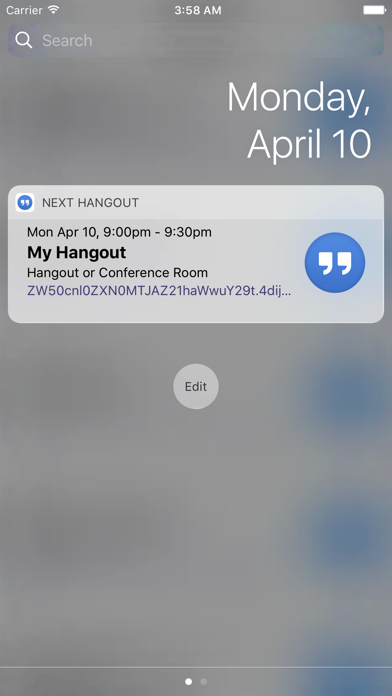The image showcases a smartphone app, focusing particularly on its home page. At the top, the status bar indicates the carrier, with the time displayed as 3:58 a.m., and a full battery icon. The date is Monday, April 10th, also shown at the top.

In the center of the screen, there's a calendar entry titled "X Hangouts," scheduled for Monday, April 10th from 9:00 p.m. to 9:30 p.m. This event is labeled as "My Hangout" and below it, the location is specified as a conference room. The address of the conference room is provided, and to the left of this information are two quotation marks.

Further below, there is an option to edit the event details. The background of the app screen is grayed out and slightly opaque, revealing indistinct blue and dark shapes. At the very top of the image, a search bar is visible. A small notification bubble is present near the bottom of the screen.